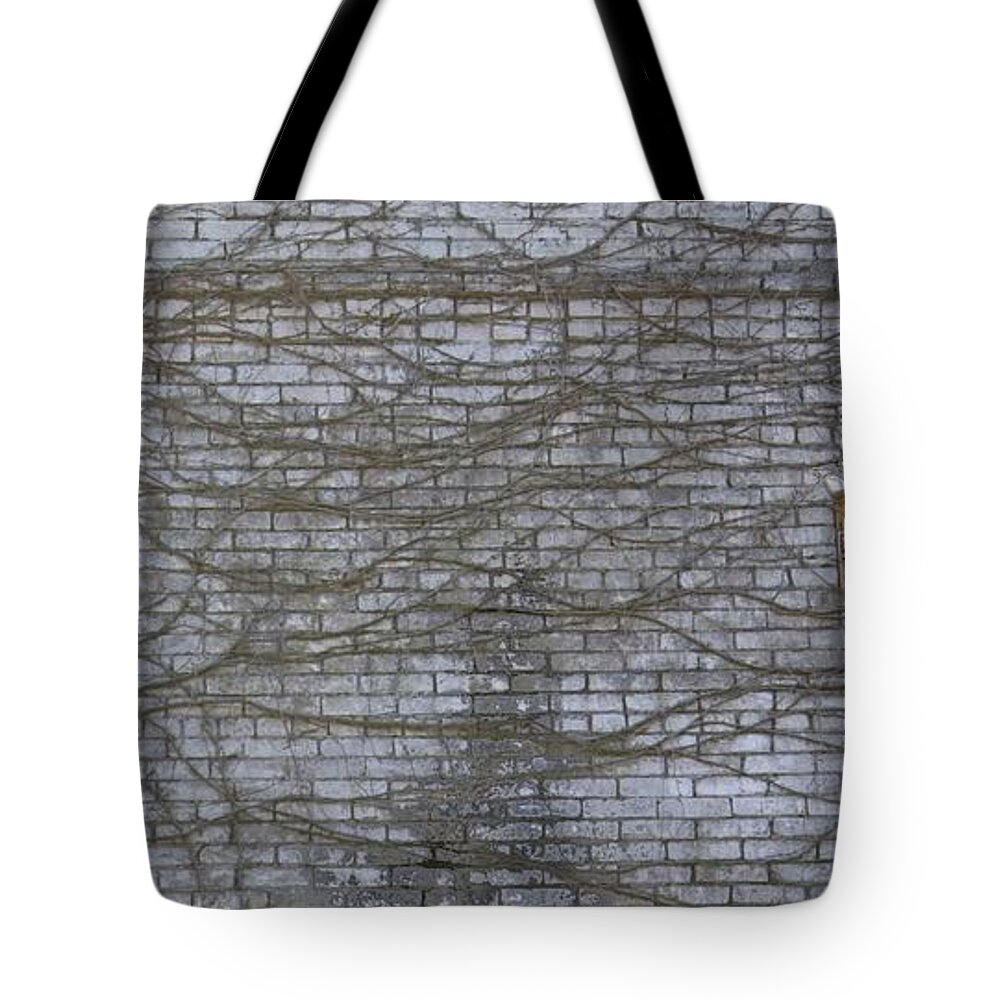This image features a roughly square-shaped tote bag displayed flat against a white background. The bag's primary color is gray, designed with a detailed brick pattern that gives it an aged, weathered appearance. The brick design varies in shades of gray, creating an illusion of old, dilapidated brickwork, much like the façade of an abandoned building. Overlaying this brick pattern are slender, root-like vines or foliage that stretch across the surface, adding an element of natural decay and roughness. The bag is equipped with a black strap handle at the top, though the strap is partially cut off in the image. This detailed, textured tote bag combines an urban, worn brick motif with organic elements, all showcased clearly against the stark white background.